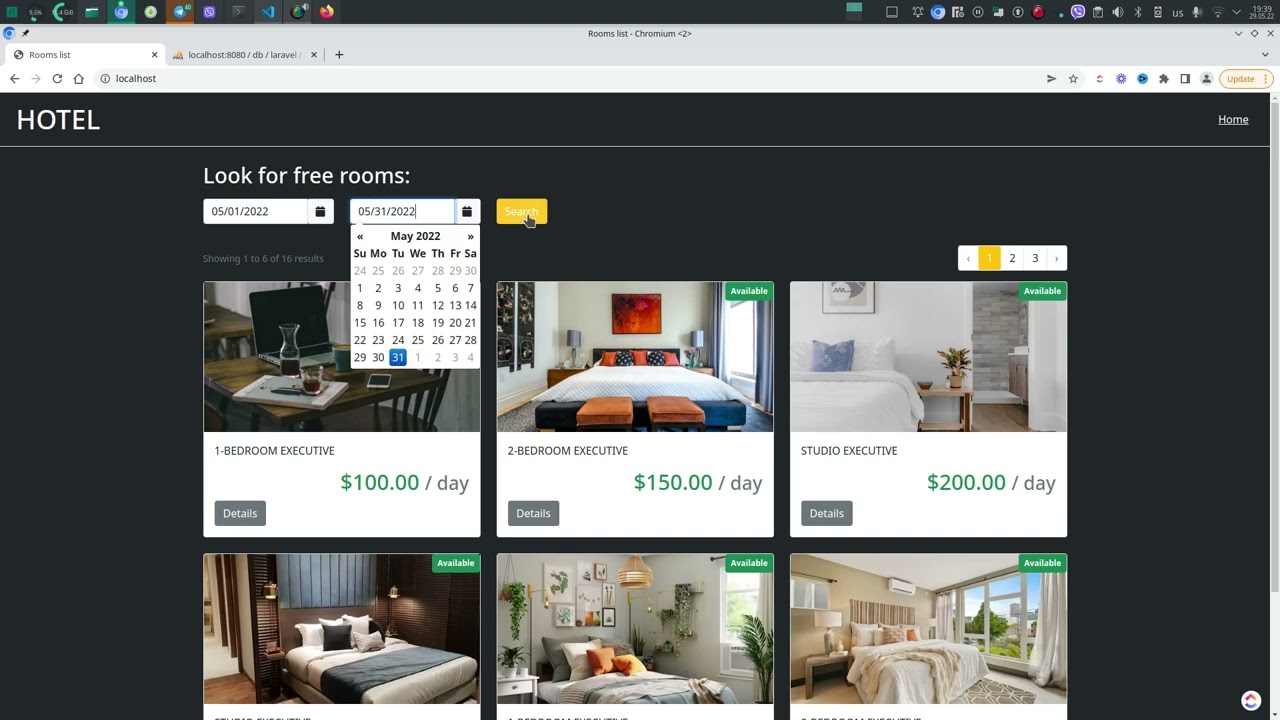This screenshot captures a desktop view featuring a booking website, with the user's taskbar prominently displayed at the top of the screen. The taskbar itself is black and cluttered with various icons, the only recognizable one being the Firefox browser icon.

At the core of the screenshot lies the booking website. The page is divided into clearly defined sections. At the top of the site, a grey tab bar shows two open tabs and a plus sign for adding new tabs, though the tab titles are indecipherable.

The website's header features the word "Hotel" in bold white block letters aligned to the left, while "Home" appears in smaller letters to the right. A white bar beneath this header segment separates it from the main content.

Below the header, the website prompts users to "Look for Free Rooms." This section includes two date selection boxes. The left date box displays "05-01-2022," and the right date box shows "05-31-2022." A drop-down calendar associated with the right date box highlights the 31st in blue. Positioned to the right of the second date box is a yellow "Search" button with white text.

Further down, a message reads "Showing 1-6 of 16 results," with six visible images of hotel rooms displayed below. The first room, labeled "1 Bedroom Executive," is priced at $100 per day and includes a "Details" button in the lower-left corner. The second room, "2 Bedroom Executive," is available for $150 per day and also features a "Details" button. The third room listed, "Studio Executive," costs $200 per day and follows the same layout with a "Details" button.

The bottom row showcases three additional hotel rooms, though the descriptions are not visible. The first of these rooms features a white bed with a dark grey runner, surrounded by dark brown, earthy tones. The middle room appears cluttered, adorned with four cushions, plants, and picture frames against white walls, giving it an open ambiance. The final room contains a white bed with a decorative throw, cream walls, and an expansive window wall on the right, contributing to a spacious feel. The overall background color of the website presents as black or dark charcoal grey, adding a sleek, modern touch.